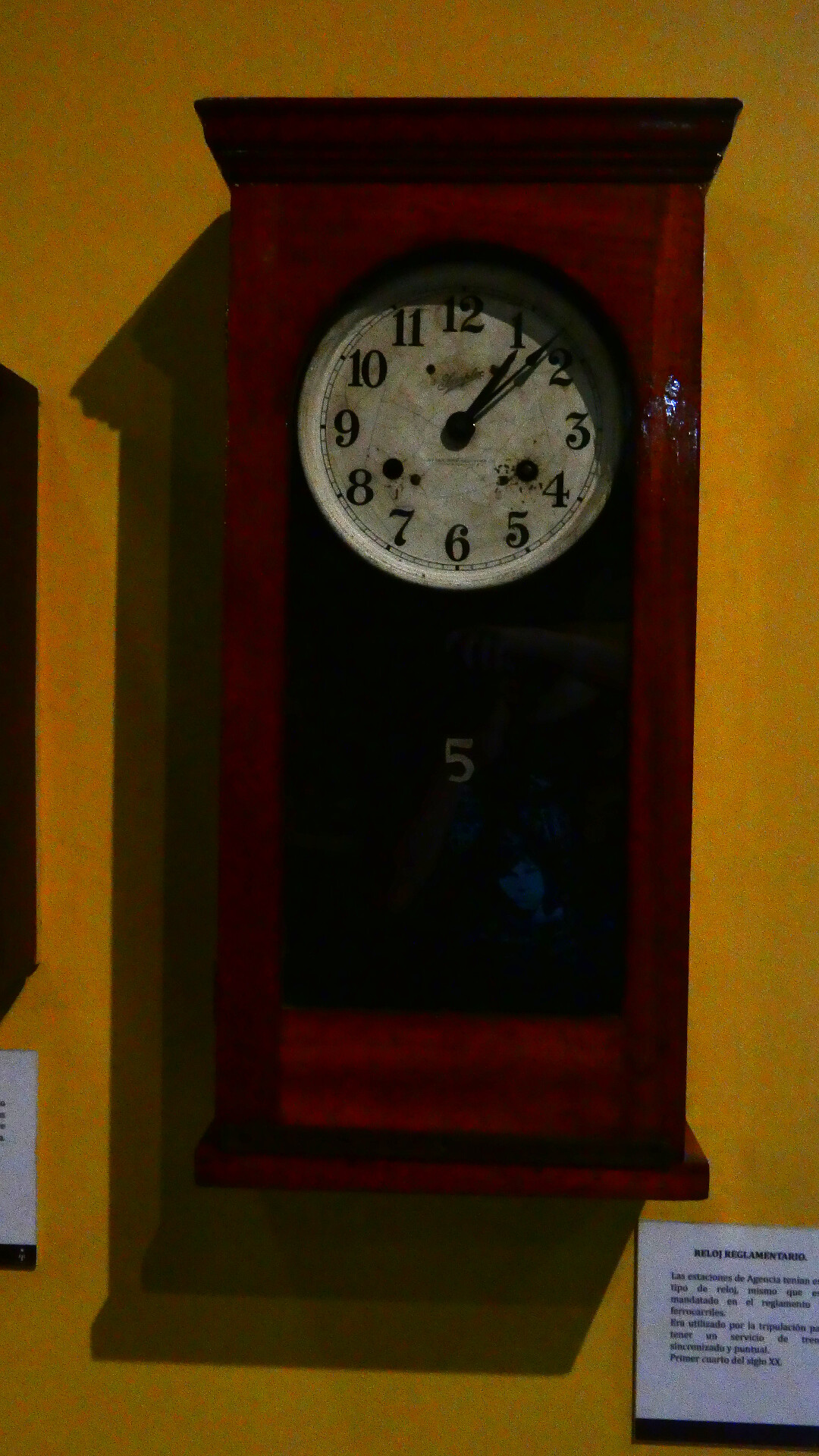The photograph features a small, rectangular wall clock with a wooden mahogany frame, hanging prominently on a yellow wall. The wooden frame appears shiny and refined, while the top portion encloses a round clock face encased behind a glass panel. The clock face, originally white, is now weathered and yellowed with age, exhibiting black and brown spots that could be rust or stains. It displays large black numbers ranging from 1 to 12 and has two black hands indicating the hours and minutes. Just beneath the clock, there's a white placard with black text, characteristic of museum displays, though the writing is indecipherable due to the image's darkness and blurriness. To the left of the clock, barely visible, is the edge of another object and another white placard, suggesting a continuation of the display. There is also a shadow of the clock cast on the wall, enhancing the depth and setting of the photograph in what seems to be a curated environment.